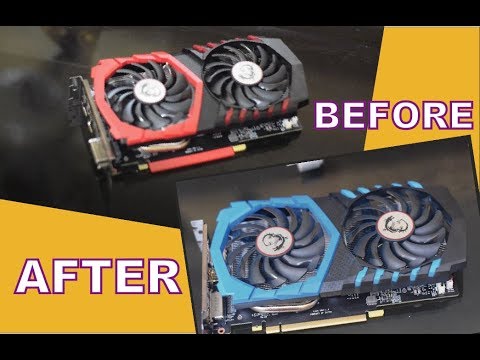The image is a horizontally oriented graphic with black bars at the top and bottom, framing a central black background. There are two photos within the graphic. At the top right, an orange rectangular area with white font reads "before," and at the bottom left, a similar orange box with white font reads "after." In the "before" section, there is a computer component, likely a cooling fan system, featuring two fans housed in black plastic with a logo in their center and red plastic surrounding them. Beneath the fans, circuitry is visible. The "after" section displays the same computer component, but the red plastic housing has been changed to a sky blue. The fans, logo, and underlying circuitry remain identical between the two images, with the only noticeable difference being the color of the plastic housing.